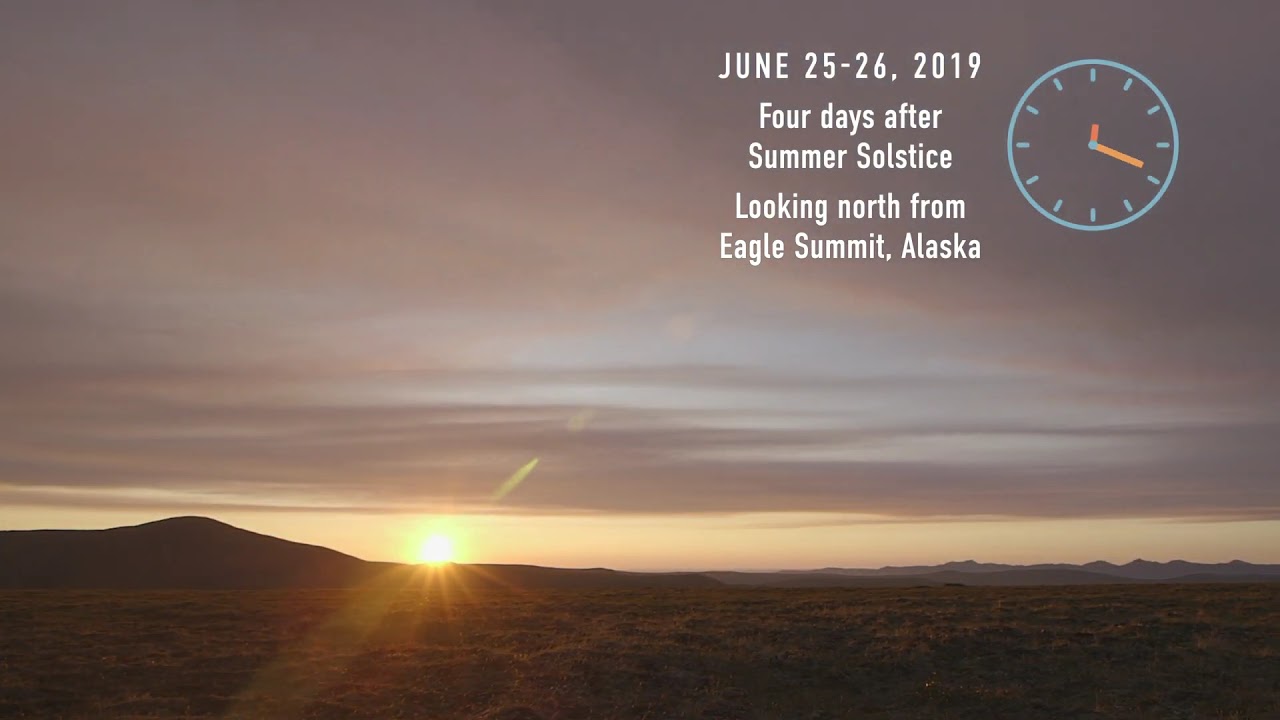Photographic landscape image taken outdoors, showcasing a dramatic sunset from Eagle Summit, Alaska, on June 25th to 26th, 2019, four days after the summer solstice. The sky, occupying the upper 60% of the image, transitions through shades of gray, blue, purple, and hints of orange. The sun, a bright yellow circle, peeks over the horizon on the lower left, silhouetting a foreground of dark land. On the right side of the image, a stretch of plains extends to distant lower mountains at the bottom right. Meanwhile, wispy clouds with purplish tints streak across the sky. A graphic of a clock in the upper right corner shows the time as 12:20, with the hour hand in red and the minute hand in orange. The caption reads in white text: "June 25-26, 2019, four days after summer solstice, looking north from Eagle Summit, Alaska."